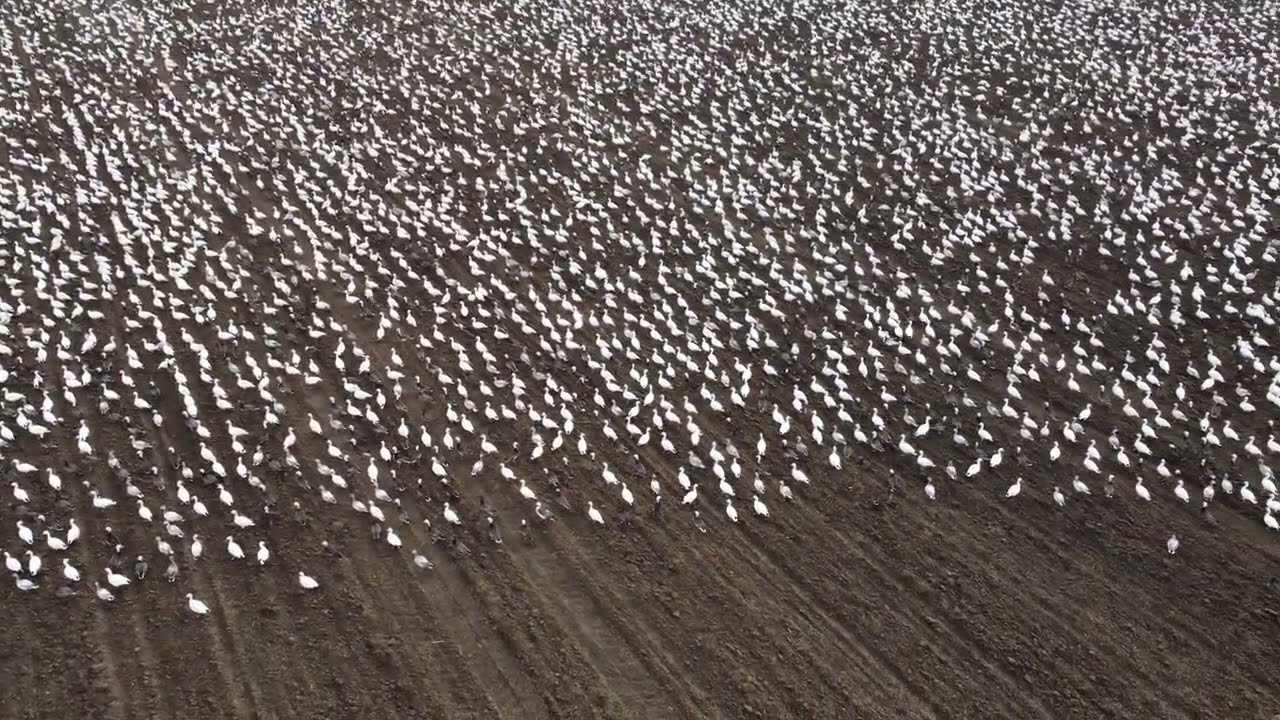In this expansive outdoor photograph, we encounter a vast, tilled, and well-maintained dirt field, possibly part of farmland, imprinted with striations that suggest it has been flattened or prepared by machinery. The field hosts an immense flock of white birds, numbering in the thousands, stretching across the majority of the image, particularly concentrated in the top 80%. The birds are small and uniformly white, with a few displaying brown feathers and white heads, possibly hinting at a diverse mix of species such as gulls or ducks, though specific identification is challenging given the distance of the shot. The entire scene is devoid of greenery, emphasizing the stark contrast between the specks of white birds and the brown, earthy background, under the clear, likely midday sky. The birds are densely packed and appear to be moving in unison, creating a dynamic yet harmonious visual of nature's congregation.